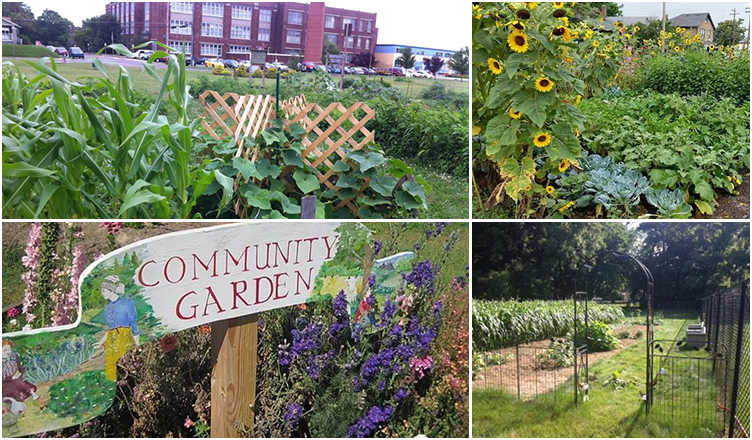This collage depicts a vibrant community garden, likely maintained by students from a nearby school. The images are arranged in a grid, with the left images being larger than those on the right. In the upper left quadrant, a large red building with numerous windows, probably a brick structure, stands in the background surrounded by parked cars and trucks. In front of it, rows of corn and vine plants ascend a wooden trellis.

To the right, in the upper right corner, another garden segment showcases tall sunflowers and various smaller plants, set against the backdrop of an older building, possibly a house. Below these, in the bottom right, the garden's entrance is displayed with a low metal fence and an arched trellis enveloped in greenery. A storage bin is visible along the fence line, and a wooded area lies behind the garden, adding a natural boundary.

The bottom left quadrant features a colorful sign that reads "Community Garden," adorned with a mural of a woman, a child, and a goose amidst garden scenery. Surrounding the sign are blooming purple and pink flowers, adding a touch of vivid color. This collage, rich with greenery and artistic elements, encapsulates the essence of a thriving community garden space.